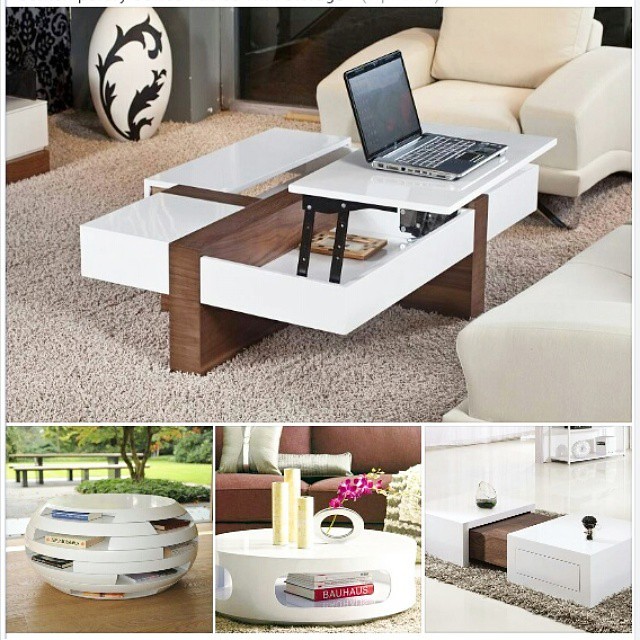This collage of four images appears to be from a professional interior design catalog, showcasing modern and stylish furniture pieces. The top image features a contemporary lounge living room. It includes sleek white leather chairs arranged around a sophisticated coffee table with a white metallic outer rim complemented by wooden inserts. A laptop rests on this table, which has a clever design allowing parts of it to lift up, supported by black metal legs. The setting is completed with a cream-colored carpet, a decorative ceramic vase with a swirling black thorn design, and a small white armchair.

The three images below present various innovative coffee tables. The bottom-left picture highlights an outdoor round coffee table seen in close-up, with segments cut out to hold books, and a solid white laminate top. The background shows grass, a tree, and what might be a bench, symbolizing an outdoor relaxation area.

The bottom middle image focuses on another round, modern coffee table with built-in shelving for books and knickknacks. It features tall white candles and a round white vase with pink flowers on top. A dark pink sofa adorned with throw cushions can be seen in the background, implying an indoor setting with a cozy atmosphere.

Lastly, the bottom right image depicts a rectangular coffee table designed with two white laminate blocks separated by a wooden insert, reminiscent of a detachable game controller. This table rests on a beige throw rug with white flooring visible behind, briefly touching on the concept of modular and easily movable furniture pieces. A small glass candle pot and a tiny ornament embellish its surface, ensuring the table's modern aesthetic stays true to form.